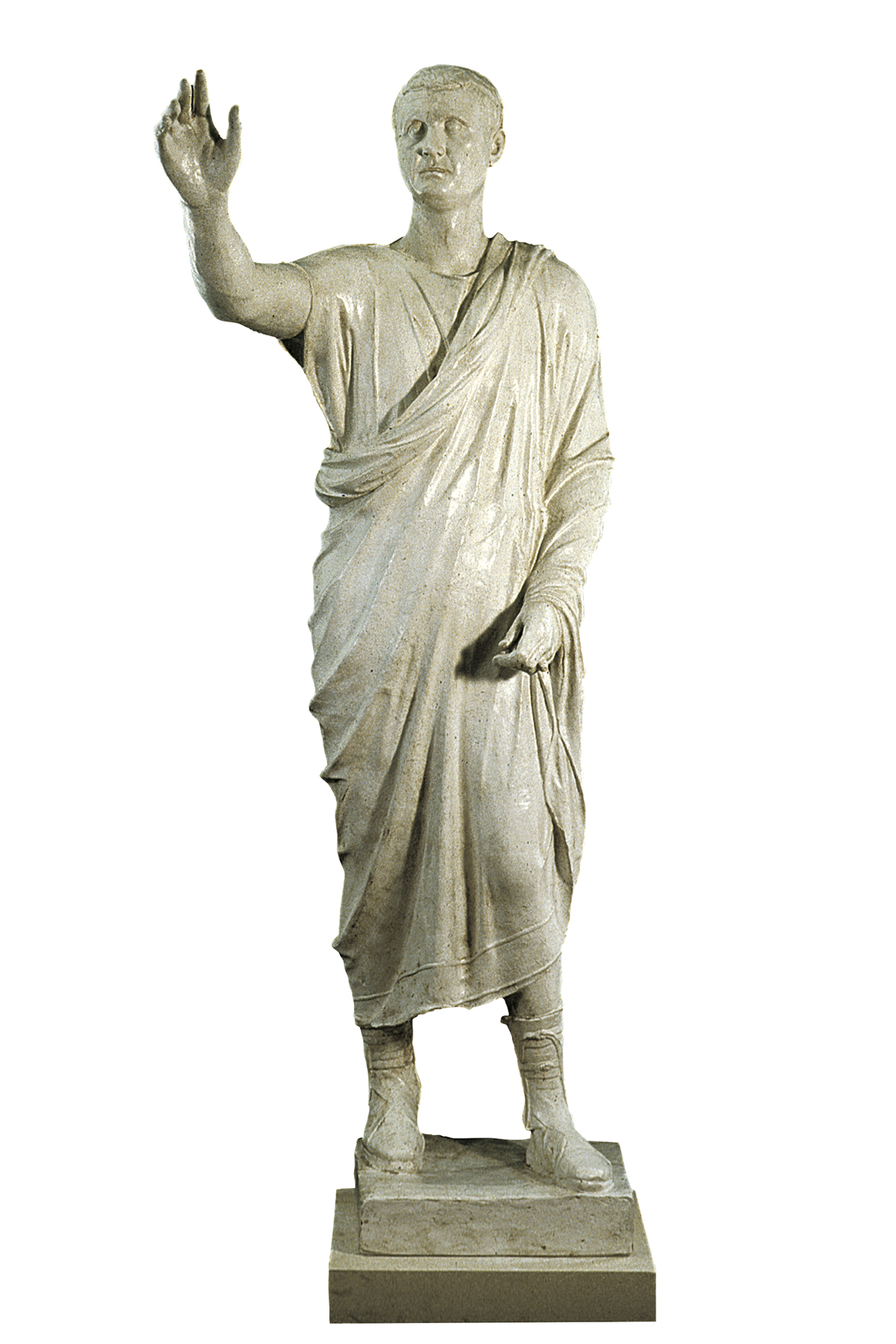The image depicts an imposing Roman stone statue, rendered in shades of off-white, gray, and black, with a slightly shiny appearance. The statue portrays a man dressed in a traditional toga draped over one shoulder and extending down to one hand. His right arm is extended outward, while his left arm remains at his side. The figure is clad in what appear to be historical leather boots and stands with a serious expression on his face. The statue is mounted on a large stone block, itself resting upon another stone block, which serves as its pedestal. The background is plain white, suggesting the setting could be a museum, with no additional elements in the frame.